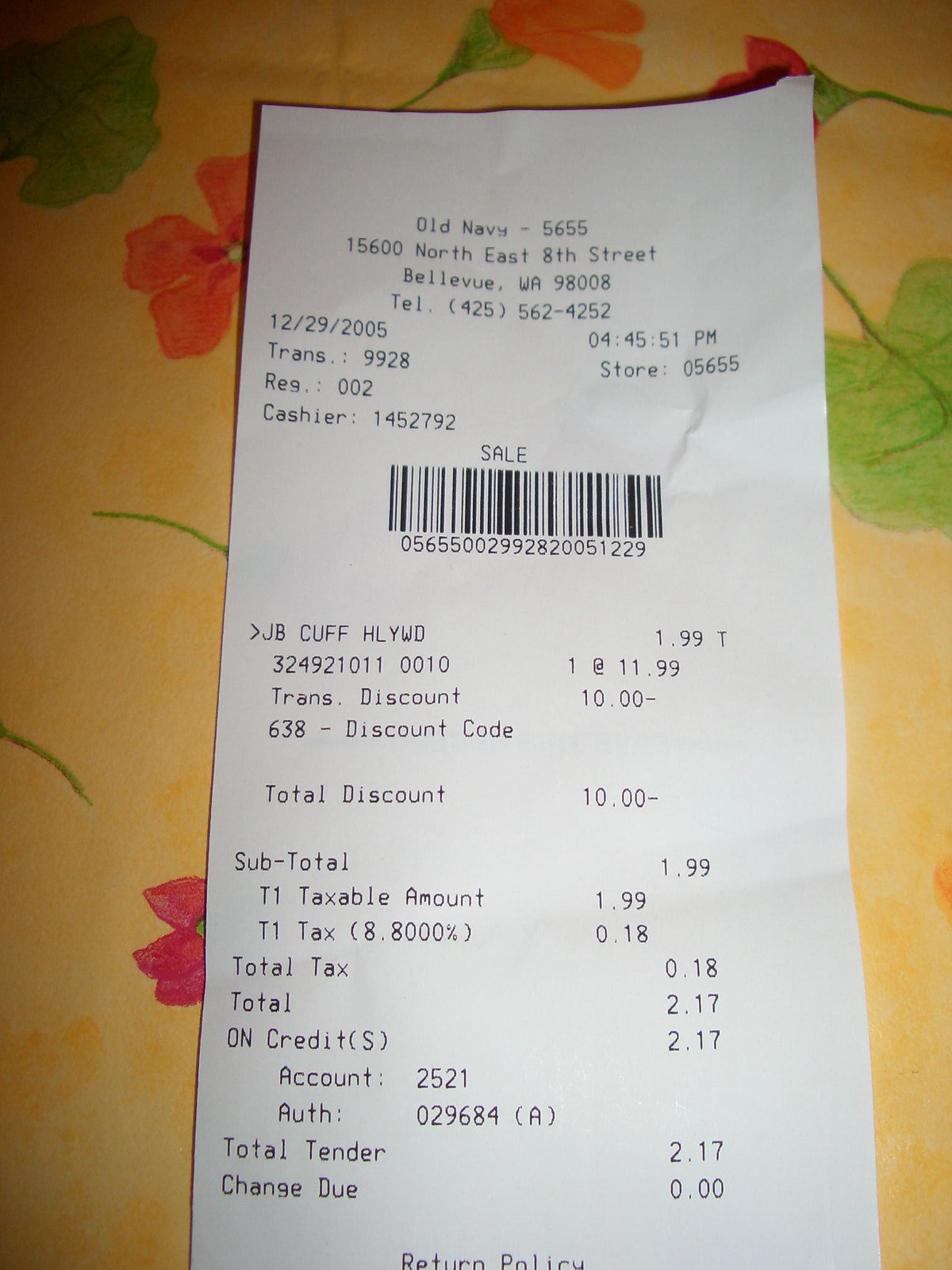A vibrant scene showcases a yellow tablecloth adorned with an intricate floral pattern featuring red and pink blossoms and large green leaves. In the background, there's a greenish-hued bottle complementing the lively table setting. Prominently displayed is a white receipt from Old Navy in Bellevue, Washington, dated December 29, 2005, with a timestamp of 4:45:51 PM. The receipt details an item originally priced at $11.99, with a $10 discount applied, bringing the cost down to $1.99. The remaining text on the receipt is rendered in clear black ink.